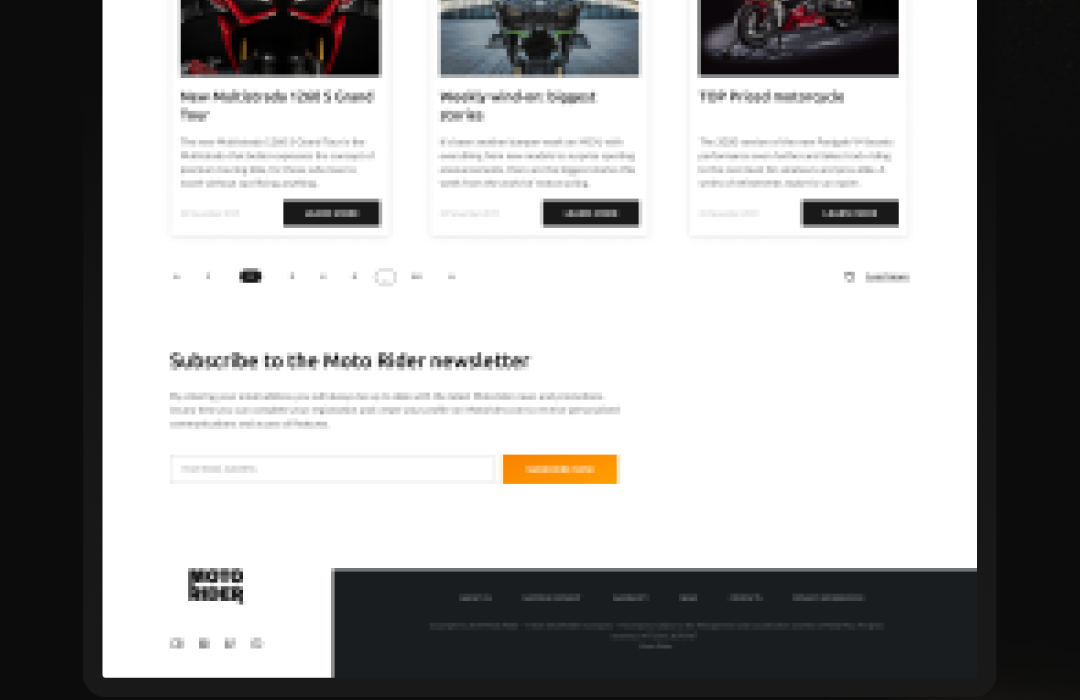This is a screenshot of a webpage with a distinctive black border on the left, right, and partially at the bottom. The bottom black border is partially obscured by a white overlay that intrudes from the main page content. The text in the obscured area is white but blurred and unreadable. The main white section of the page features a prominent, elongated hook-shaped design that dips lower than the rest of the content. 

At the top of the main section, there are three square panels, each containing an image with some small, difficult-to-read text beneath them. Below these images, there is a dark rectangular button intended for purchasing or progressing to the next page. 

Further down, a call-out section invites users to subscribe to what appears to be the "MoboRider" newsletter. The subscription form includes a field for entering an email address and an adjacent button—either blue or orange with white text—to finalize the subscription. Additional text presumably providing more details about the newsletter is present but remains unreadable.